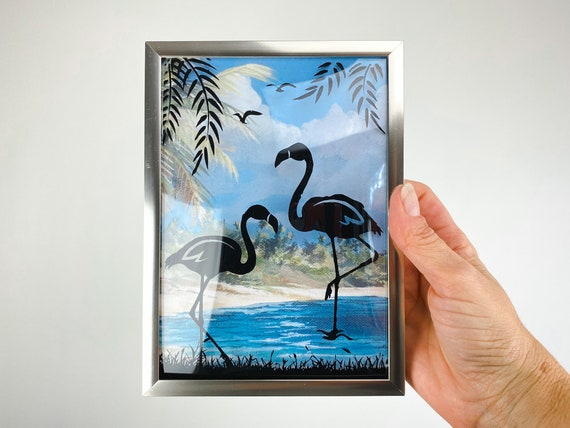In this image, we see a man's right hand holding a picture framed in a silver-colored frame, situated near the bottom right corner and centrally within the image. The background is a very light gray. The picture within the frame is a colorful outdoor scene featuring two silhouetted black flamingos or cranes with long curved necks and long legs, one of which is raised as if walking. The birds are standing in a shallow pond of blue water, where their feet are visible. The surrounding environment includes a sandy beach area with brown and cream tones, dotted with vegetation and shrubbery. Above, the sky is blue with some clouds, including thunderclouds, and a couple of seagulls flying. Branches with leaves and fronds frame the top edges of the scene, creating a naturalistic border.